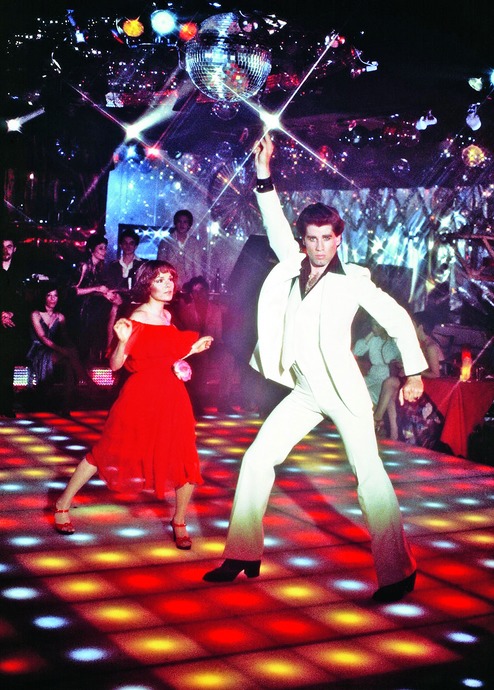The image captures a vibrant, realistic scene from the iconic disco-era movie "Saturday Night Fever," starring John Travolta. Set on a multicolored, illuminated dance floor with checkered patterns of orange, red, and white squares, the photograph highlights Travolta in a classic 70s white suit that features a distinctive black triangular collar. He strikes an exuberant disco pose with his right arm pointing upwards, his feet pivoted, and his gaze fixed confidently ahead, capturing the essence of the era's dance style. His outfit is complemented by tall, black platform boots and a partially unbuttoned black shirt revealing his chest. To his left, a woman—presumably his dance partner—dressed in a flowing, knee-length red dress and matching red high heels, looks toward him, engaged in the lively moment. Above them, a silver disco ball radiates sparkling lights across the room, adding a magical brilliance to the nightclub atmosphere. Around them, other club-goers watch from tables and along the walls, enveloped by the shimmering, colorful lights. This scene is iconic for its feeling of vibrant energy and captures the quintessential disco nightlife.